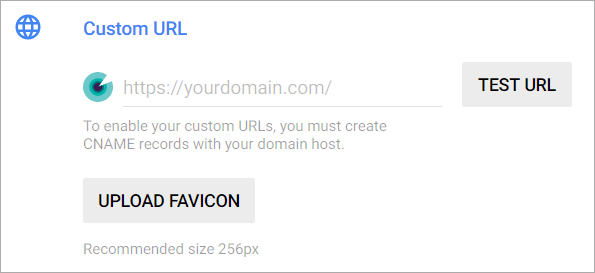The image is a screenshot displayed in landscape mode, bordered by a very thin light black line. The screenshot itself has a completely white background. In the upper left corner, there is a blue globe icon featuring two horizontal lines and two curved lines extending from north to south, all enclosed within a blue circle. Adjacent to this icon is the text "Custom URL" in blue, which appears to be non-clickable and merely styled in blue for emphasis.

Beneath this section, there is a form where users can input their information. A green icon is displayed, resembling a black dot at its center with a pie-slice-shaped white cutout. The surrounding area of this icon features various shades of green. Below the icon, a light gray line is slightly difficult to read against the white background. This line contains the placeholder text "https://yourdomain.com/" indicating where users should enter their full URL.

To the right of the input field, there is a gray button labeled "Test URL" in dark black text. This button likely functions to check the availability or validity of the entered URL. Underneath this section, additional instructions are provided in gray text, stating "To enable your custom URLs, you must create CNAME records with your domain host." 

Further down, there is another gray button with dark black text labeled "Upload Favicon," followed by the note "Recommended size 256px."